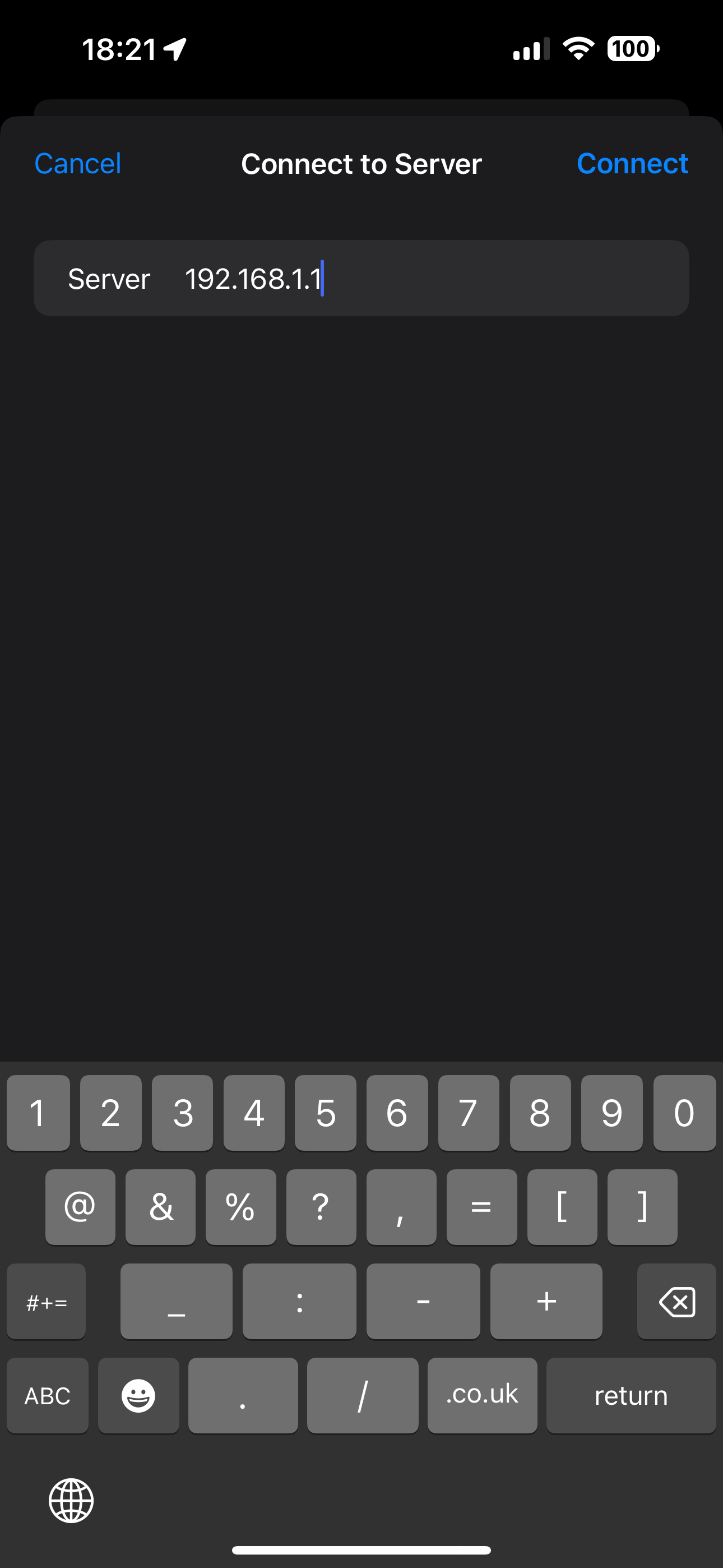Screenshot of a Cell Phone Screen Attempting to Connect to a Server

The image shows a vertically-oriented, slightly compressed screenshot of a cell phone screen. The background is predominantly black, enhancing the contrast of the foreground elements. At the top left, the time is displayed as "1821" (or 6:21 PM in 24-hour format). In the top right, indicators show a full battery, signal strength, and data connection status.

Central to the image, in large white font, is the prompt "Connect to Server," suggesting the purpose of the screen. To the left of this prompt, in blue text, is the option "Cancel," while to the right, also in blue, sits the option "Connect." Below this, there is an input box, slightly lighter in color than the black background, displaying the server address "192.168.1.1" in white font, with a vertical blue cursor line positioned at the end of the text.

The lower portion of the image is dominated by a virtual keyboard set to numbers and special characters mode. The top row contains the numbers 0 through 9, the middle row includes various symbols, and the bottom row comprises mathematical operators like minus and plus.

Overall, the image clearly depicts an active attempt to connect to a server via a cell phone.